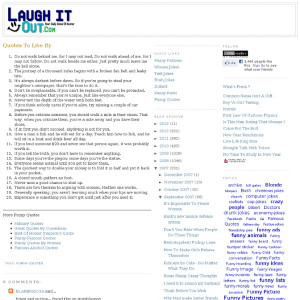A small, low-resolution screenshot captures a 4:3 aspect ratio snapshot of a vintage website named laughitout.com, which features a collection of humorous quotes, jokes, and anecdotes. Due to the image's poor quality, much of the text is barely readable or completely illegible. The webpage is set against a white background with dark text. On the bottom right side, there's a word cloud of hyperlinks that highlight the recency and frequency of certain topics. The laughitout.com logo is prominently displayed with "laugh" and "it" in dark blue, "out" in a lighter blue, and "dot com" in bright green, all in bold block letters. Below "laugh" and next to "out," a smiley face adds a playful touch. Although the website seems to have a tagline, it is indiscernible due to the image’s resolution. The design suggests an old-school aesthetic, reminiscent of early Blogger or WordPress platforms, indicating that the screenshot might capture an earlier version of the site.